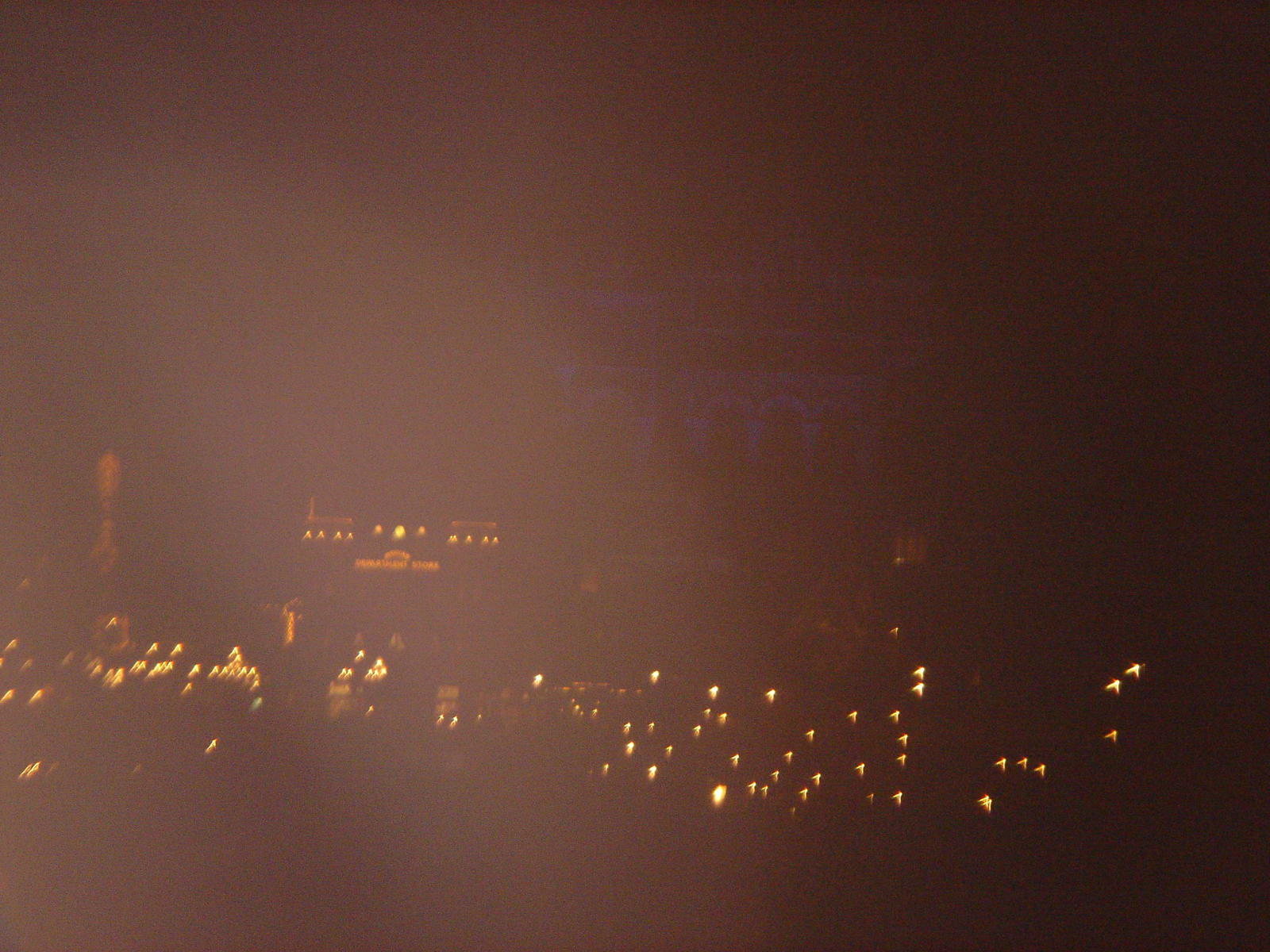This nighttime photograph is characterized by a hazy, out-of-focus appearance that blurs the details, giving it a blackish-white, grayish ambiance. The image is largely dominated by darkness, with scattered, tiny specks of light appearing unevenly throughout. These lights could be coming from various sources—possibly candles, streetlights, neon signs, or illuminated windows from buildings. There is a particularly prominent faded source of artificial light in the bottom left corner that seems out of place, adding to the enigma of the scene.

The overall scene suggests a cityscape, potentially viewed from a distance or an elevated position, where large buildings, perhaps a temple, a government structure, or even an aqueduct, loom in the darkness. The lights appear to follow a logical arrangement, indicating streets lined with buildings, possibly even showing hints of moving cars and neon signs. One building, in particular, seems to be partially identifiable by orange illuminated letters and rows of lit windows, though the poor focus and overexposure obscure the finer details.

The photograph’s unclear clarity and overexposure result in a mixture of light and dark, creating a visual puzzle of lights and shadows set against the nighttime backdrop.